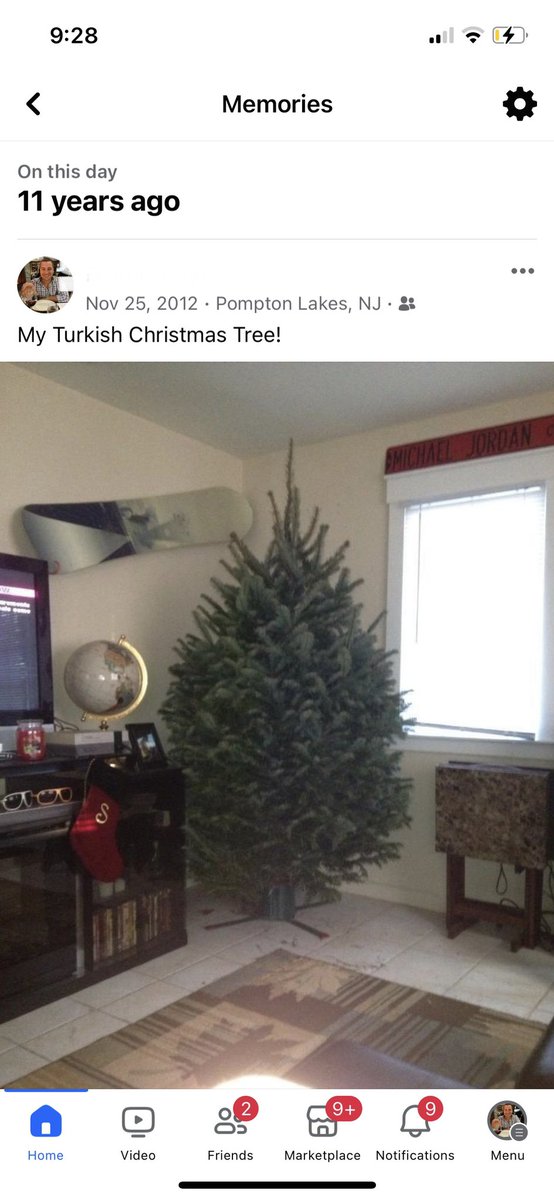Screenshot Caption: 

This detailed screenshot captures the "Memories" page on the Facebook mobile app. The device's time is displayed at the top left corner, showing 9:28 AM. Adjacent to the time, the top right corner features various phone icons indicating battery percentage, Wi-Fi strength, and signal status.

Centered prominently below the status bar, "Memories" is written in bold black font. To its right, a cogwheel icon for settings is visible, while a back arrow on the left allows users to navigate back to the Facebook homepage.

The main content of the screenshot highlights a memory from "On This Day 11 Years Ago," with "11 years ago" standing out in larger black font. The memory post is displayed in full detail below this heading. The post consists of a user’s profile picture (with the name edited out) at the top left, and the date and location beneath it. Next to the date, an icon indicates that the post was shared with friends only.

The post's content reads "My Turkish Christmas tree," accompanied by a large photo of an undecorated tree placed in the corner of a home. This image is the focal point of the memory.

At the bottom of the screenshot, a horizontal menu features icons representing various Facebook sections: Home (highlighted in blue to show it is currently selected), Video, Friends, Marketplace, Notifications, and the user's profile photo. The Friends, Marketplace, and Notifications icons have red circles with numbers, indicating the alerts for each section.

This screenshot captures a nostalgic Facebook memory with detailed contextual information, providing a clear view of the user's mobile interface and the specific memory being revisited.